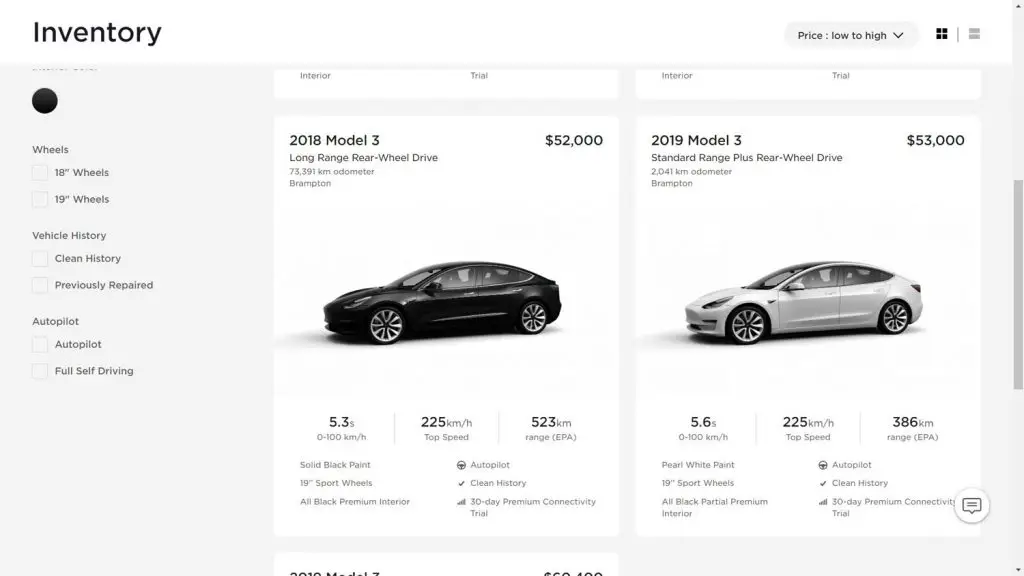Displayed is an inventory screen for a car dealership's website. At the top left corner, there is a label that reads "Inventory" in black text against a white background. Adjacent to this label, towards the right, there is an option selected for sorting the listed cars by price from low to high. 

On the left sidebar, there are several clickable filter descriptions available: "18 inch wheels," "19 inch wheels," "vehicle history," "clean history," "previously repaired," "autopilot," and "full self-driving."

Two cars are listed on the page:

1. **2018 Tesla Model 3 Long Range Rear Wheel Drive**: Priced at $52,000, this vehicle comes with solid black paint, 19-inch sport wheels, and an all-black premium interior. It is equipped with autopilot and boasts a clean history. The car also includes a 30-day premium connectivity trial.

2. **2019 Tesla Model 3 Standard Range Plus Rear Wheel Drive**: This car is listed for $53,000. It features pearl white paint, 19-inch sport wheels, and an all-black partial premium interior. Like the previous vehicle, it also has autopilot, a clean history, and includes a 30-day premium connectivity trial.

The image prominently shows the black 2018 Model 3 on the left side.